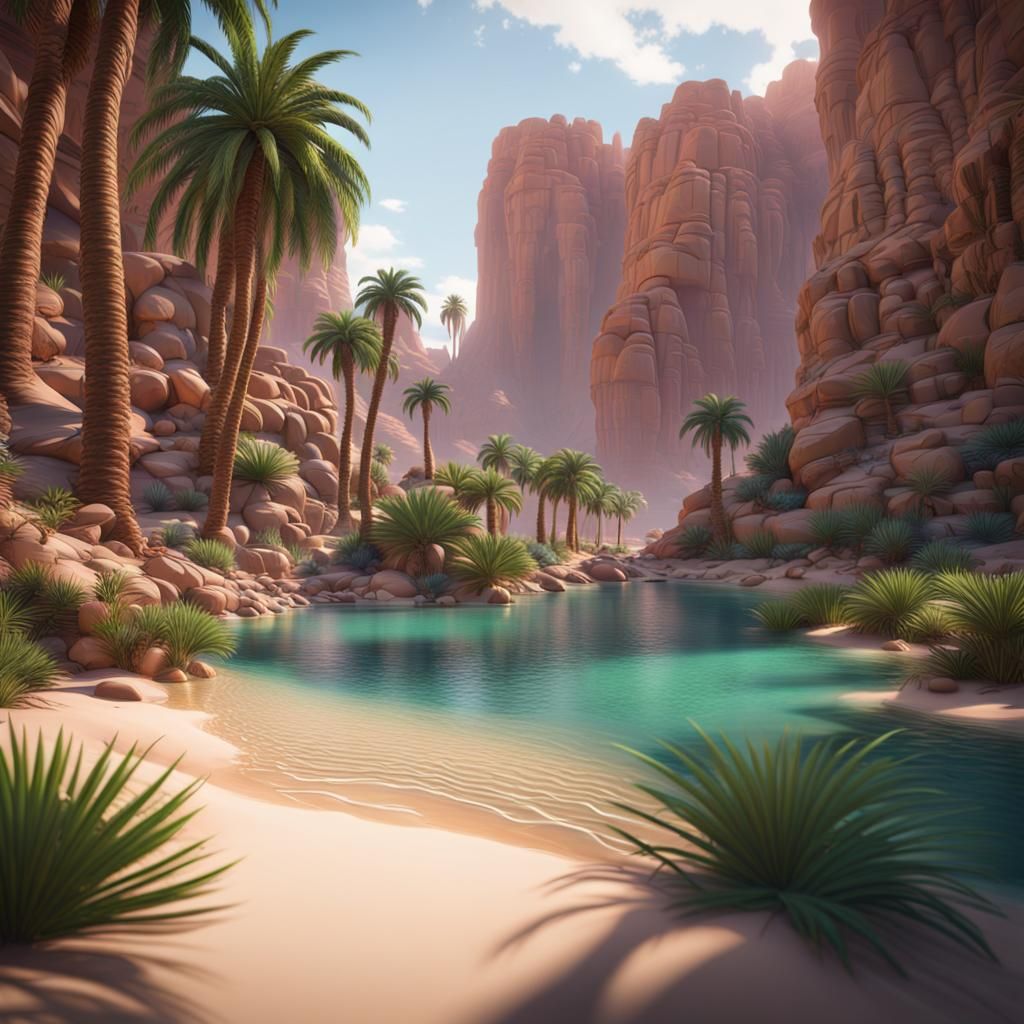The image depicts a digitally created, oasis-like scene set in a tropical canyon. The vibrant blue sky is adorned with scattered white clouds that cast subtle shadows on the landscape below. The picture showcases a narrow, meandering waterway with an aqua-green hue, occasionally darkened by shadows from towering, light-brown rocky cliffs on either side. The water rests alongside a sandy shore on the left, where lush palm trees and aloe vera plants with sharp, green leaves thrive. These trees stand tall amidst an array of scattered boulders, reinforcing the tropical essence of the valley. The entire scene is framed by the imposing rocky walls, creating a stunning contrast between the arid, mountainous surroundings and the verdant, oasis-like interior.